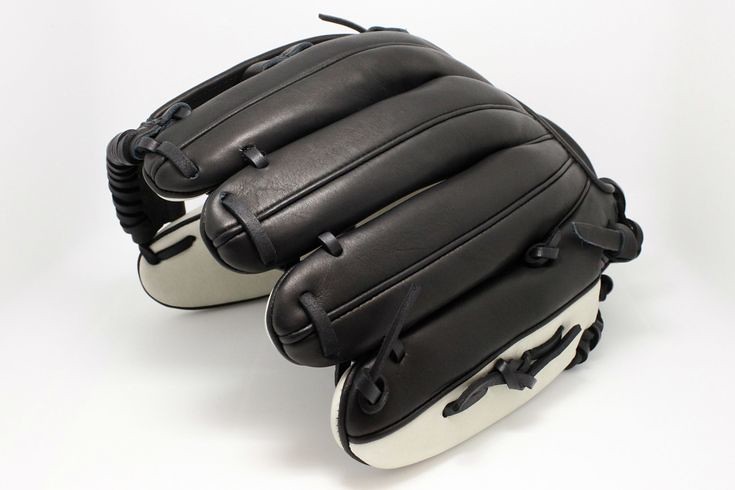In this image, there is a detailed photograph of a baseball mitt. The mitt is predominantly dark brown leather with white sections around the thumb and index finger. The top part of the mitt—the area that catches the ball—is facing upwards, showcasing its intricate design. The webbing and middle fingers of the mitt have dark brown leather straps for added reinforcement, and the base of the mitt also has black straps for a secure fit around the wrist. The glove is set against a stark white background, with a light source from above casting a faint grey shadow beneath it, adding depth to the image.